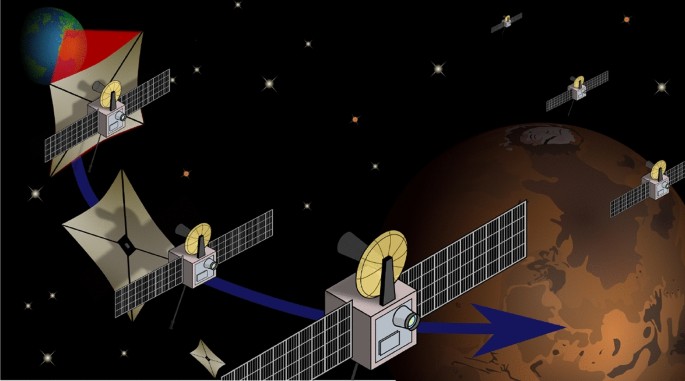The image is a detailed graphic illustration set in outer space, showcasing six satellites orbiting the Earth. In the upper left-hand corner, the Earth is depicted with a map outline highlighting the continents near the North Pole and Europe. Each satellite features black, shiny wings extended from its sides and distinct yellow, metallic-looking discs on top. The satellites are shown following a specific path, indicated by a blue arrow pointing from the first to the third satellite as they trail from the Earth toward the right side of the image. In the lower right-hand corner, Mars is illustrated in various shades of brown with three satellites hovering above it. The entire scene is set against a backdrop of deep black space filled with numerous twinkling white and reddish stars.